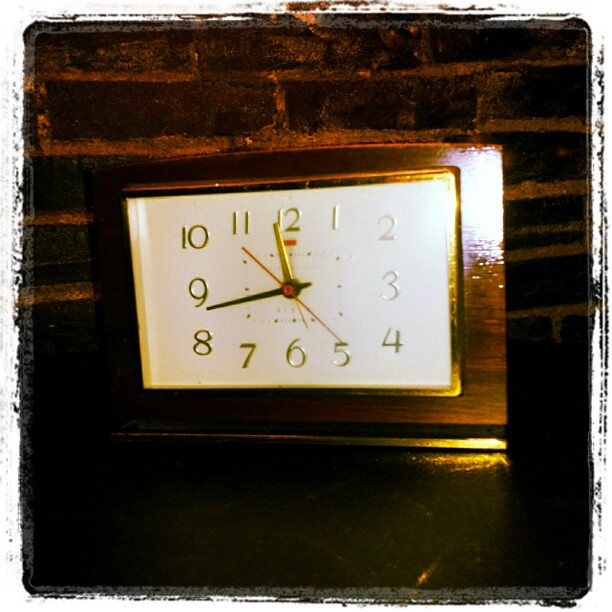An up-close photograph captures a square clock against a dark backdrop that resembles a black brick wall with gray mortar. The clock’s casing, on the right side, appears to be a reddish-orange dark wood featuring black streaks, while the left side merges seamlessly with the background, rendering its boundary almost undetectable. The clock face is also square, outlined in gold, and features a pristine white surface. The numbers adorning the clock face are gold, matching the hour hand, while the minute hand is black, and the second hand stands out in red. A strip of gold decorates the bottom of the clock's enclosing box, adding an additional touch of elegance to the overall design.